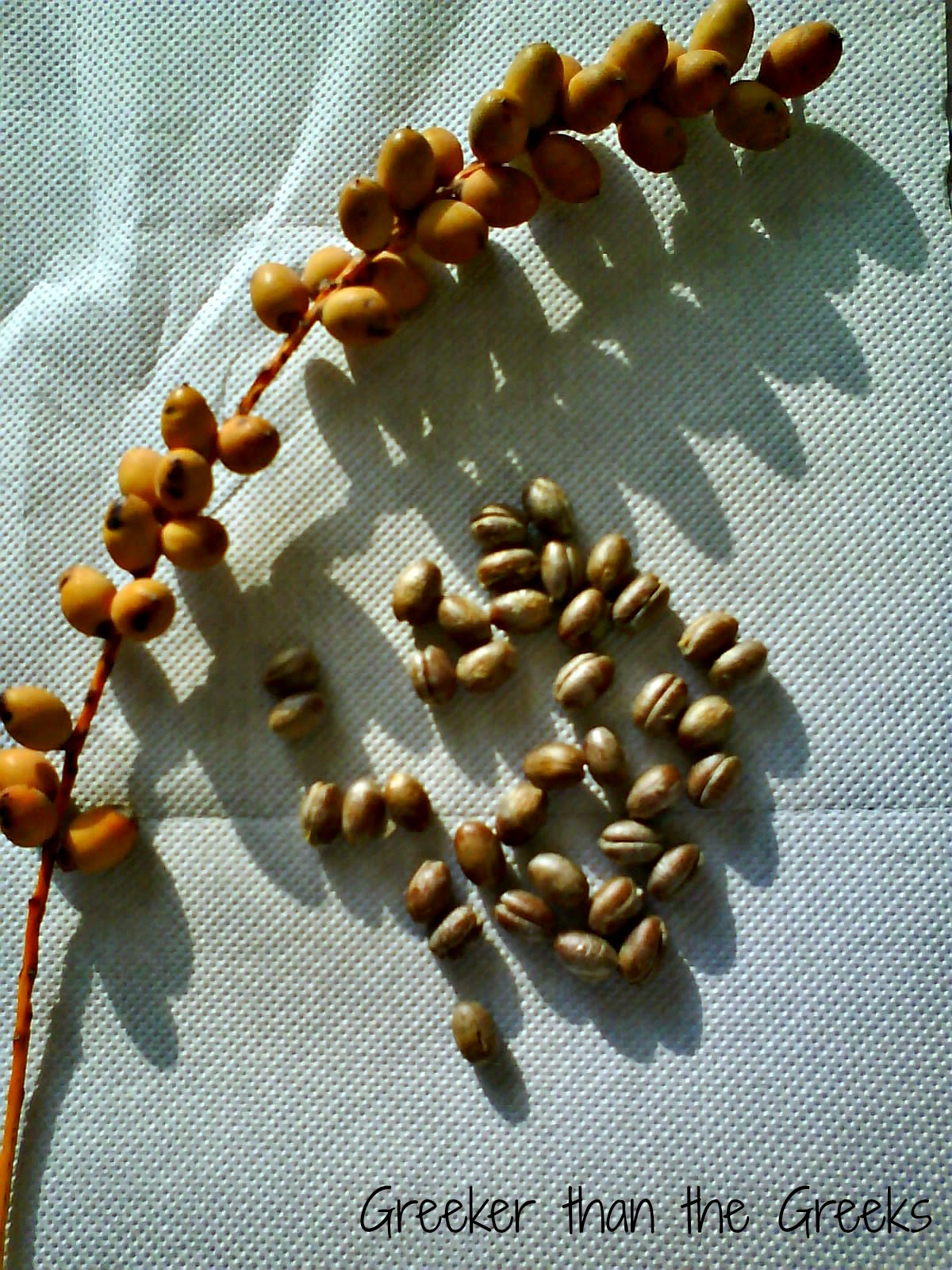The photograph features a long olive branch with several oval-shaped green olives, placed on a mostly flat white surface that appears to be paper towel or fabric, though the top left corner is wrinkled. To the right of the branch are numerous round, brown seeds resembling coffee beans. The surface under the items has many small holes. The green olives are unpicked and arranged along the branch, which stretches from the bottom left to the top right of the image. Meanwhile, the scattered brown seeds lie adjacent to the branch, concentrated around the middle. Overlaying the surface in the bottom right corner is black text reading "Greeker than the Greeks."